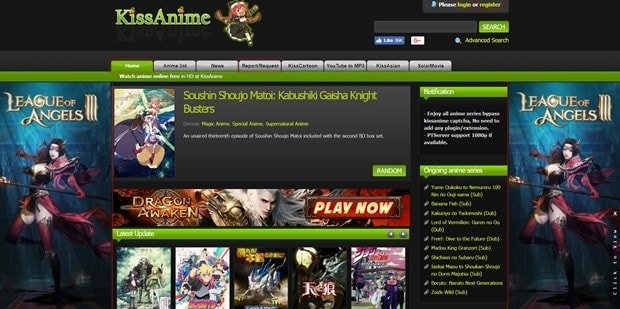A detailed screenshot caption:

"The screenshot displays a vibrant interface from the game 'League of Angels 3'. Dominating the screen is the name 'Kiss Aneem' in bold green letters. Just above, the title 'League of Angels' is prominently featured. Among the center-right details, the text 'Sushin Shuju Matoi' is visible along with 'K.A.B.U.S.H.I.K.I' and 'Ayesha Knight Busters'. On the left side, there is a green triangle labeled 'Random' and a green rectangle with white text commanding 'Play Now'. A 'Notification' icon is also present, indicating activity, and there's a hint of an 'Ongoing Aneem Series' list along one side. Flanking the screenshot on both the left and right are posters portraying an ethereal woman, tying back to the 'League of Angels 3' theme."